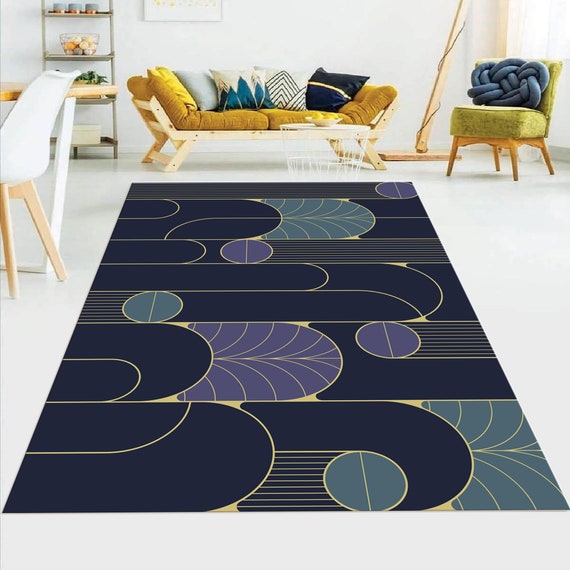This photograph depicts a modern, stylish living room with a predominantly white and natural wood color scheme. The centerpiece of the room is a large, modern-art-inspired rug featuring an array of geometric and organic patterns. The rug primarily showcases blue fields with light gold or yellow trims and purple accents. Some patterns resemble cylindrical shapes with circular tops, while others look like flattened screw head designs and large fern-like motifs.

A natural wood-framed couch, possibly pine, is positioned against the white wall, adorned with golden cushions and a mix of multicolored pillows. Adjacent to the couch, a table or basket-like object is present, possibly serving as a functional yet decorative element. To the left, a green-cushioned chair with a peculiar blue throw pillow sits on a wooden pedestal.

In the background, there are additional seating options, including a chair drawn up to what might be a dining table, suggesting a combined living and dining area. A bookshelf with various items adds further interest and utility to the space. Overall, the room balances minimalist color schemes with artistic, eye-catching elements in the rug and furnishings.